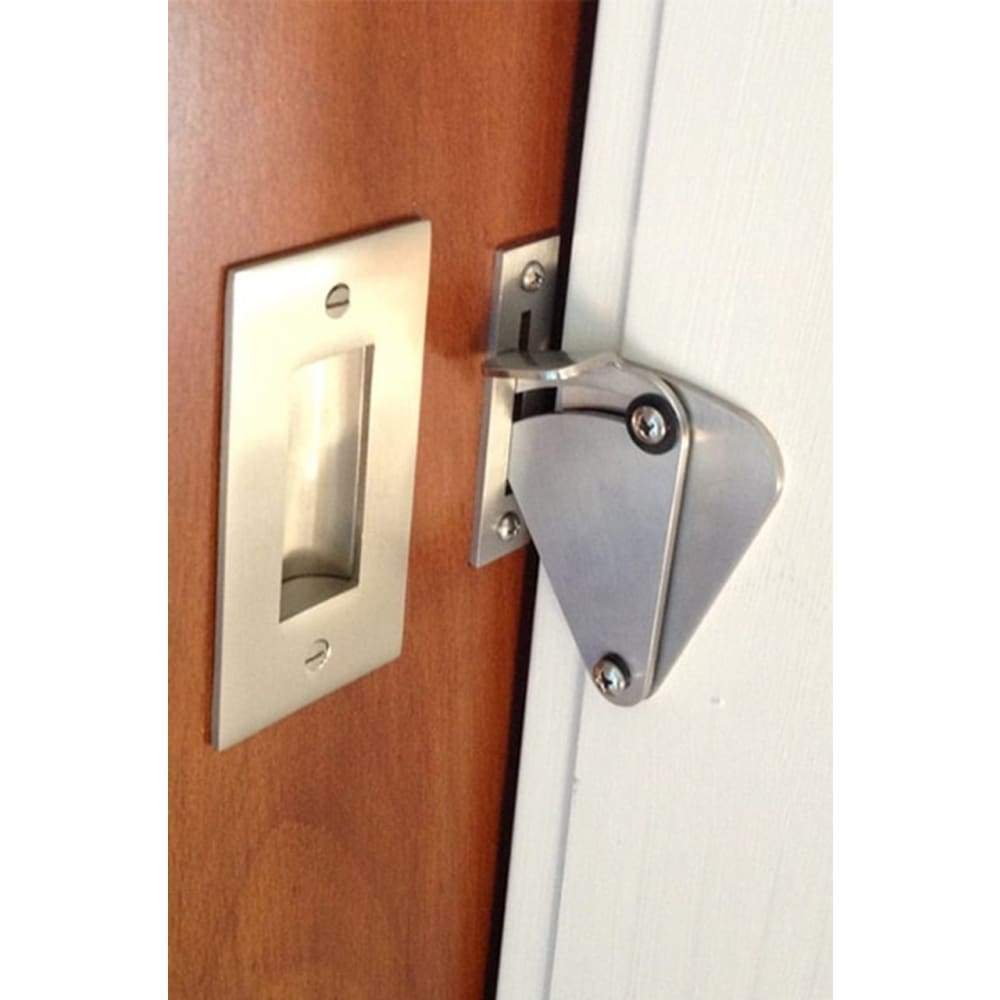The image depicts a sliding door with a lock. The door, positioned on the left side of the frame, features a handle located in the center. The lock mechanism includes a metal latch protruding from the door and fitting into a square metal slot affixed to the adjacent wall. The door is made of reddish-brown wood, while the wall to its right contrasts in white. The colors observed in the image include brownish tones, metallic gray, black, and white, suggesting a domestic setting.